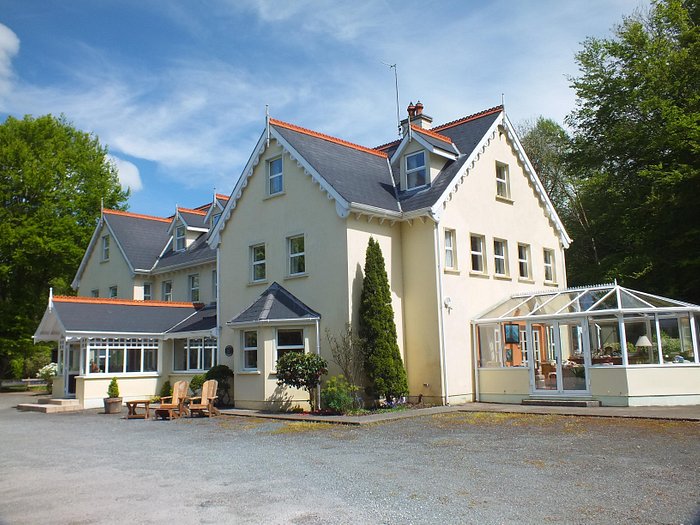This photograph captures a large, three-story house under a vast blue sky with scattered white clouds. The pale yellow house features white lattice detailing and pointed roofs, with a wing extending to the left adorned with multiple dormer windows. On the right side, there is an atrium or greenhouse-like structure with glass windows and a glass roof, filled with plants, couches, and a small lamp, creating a bright sitting area. The front entrance is accessible via two wooden steps, leading up to the house. In front, there's a mix of small bushes and tall, tree-shaped hedges. Two Adirondack chairs are positioned on the gray asphalt or gravel area before the house. Deciduous trees frame the scene on both sides, enhancing the picturesque setting.